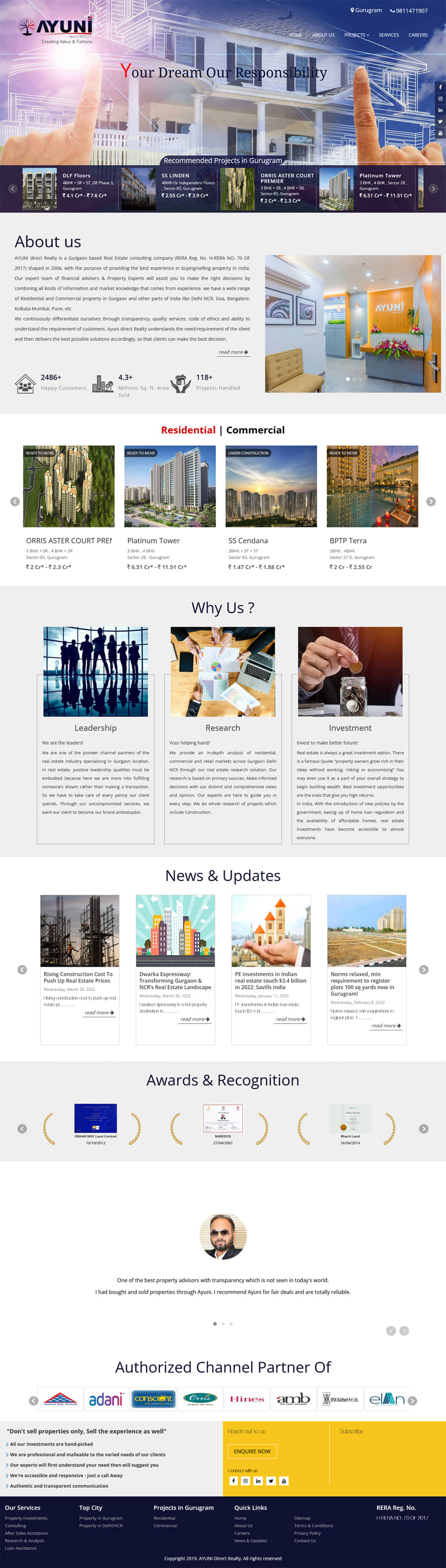Here is a detailed and polished caption for the described image:

This image is a cropped screenshot from a commercial or residential architecture company's website. At the top, there is a visually striking photo background that showcases the front facade of a modern house. The photo dramatically transitions from the constructed left side of the house to a blueprint of the right side, illustrated by a person's hand pointing at the blueprint. Beneath this, a light gray section prominently features the heading "About Us" in a large, bold gray font, accompanied by a descriptive paragraph.

To the right, there's a large square photograph depicting the company's office environment. Below this, there are four thumbnail images showcasing various completed architectural projects. Further down in the center, another large gray section with the text "Write Us" takes precedence.

Continuing below, three boxes are neatly arranged, each with a thumbnail image at the top and a corresponding description beneath it. Following this section, the website highlights a "News and Updates" area featuring four distinct story icons.

Toward the bottom, in a gray section labeled "Awards and Recognition," three icons represent different accolades the company has received. At the very bottom center, the page showcases a profile photo and a brief introduction of the company's owner. Completing the design, the top left corner prominently displays the company logo, "AYUNI."